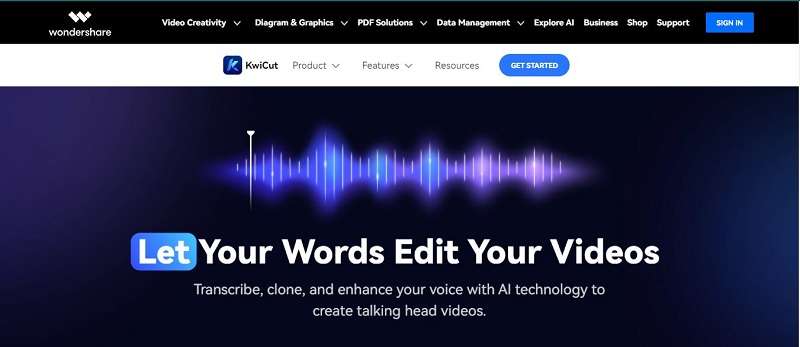The image is a rectangular, landscape-oriented snapshot from a website called Wondershare. The interface is clean and modern, featuring a prominent black menu bar at the top. Although the typical browser menu and website address are absent, the black header prominently displays the Wondershare name in white, accompanied by a sleek 'W' logo.

The menu bar includes the following dropdown options: 'Video Creativity,' 'Diagram and Graphics,' 'PDF Solutions,' 'Data Management,' 'Explore All,' 'Business,' 'Shop,' and 'Support.' Most of these menu items have pull-down options, specifically the first four. Positioned at the far right of this menu bar is a blue button with white text that says 'Sign In.'

Directly below this black band is a white band across the width of the website, displaying the text 'KiwiCut,' alongside a 'K' logo. This section also includes dropdown menus labeled 'Product,' 'Features,' and 'Resources,' followed by a blue, bullet-style button with white text that reads 'Get Started.'

Beneath this white band, the website showcases a dark blue graphic depicting sound waves in a lighter blue and white, symbolizing audio activity. Below this visual, the text reads, 'Let your words edit your videos, transcribe, clone, and enhance your voice with AI technology to create talking head videos.' This promotional message is entirely in white text, except for the word 'Let,' which is highlighted with a blue box around it.